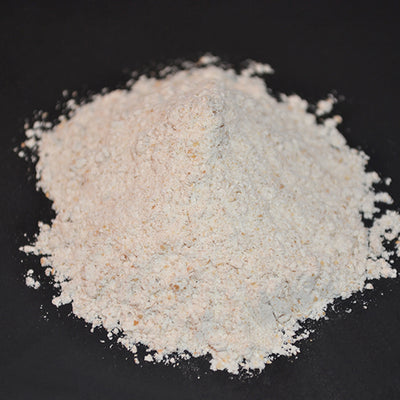The image depicts a pale, off-white powdery substance, similar in texture to finely ground grains or possibly even protein powder. This substance is arranged into a neatly heaped mound with a pointed top, though the edges slightly spread out. Mingled within the powder are tiny flecks of various colors, including yellow, orange, purple, red, and brown, possibly remnants of grain coatings or mineral inclusions. The entire scene is set against a matte black background, accentuating the central placement and fine details of the powder. The photograph is simple and devoid of any other text or extraneous elements, focusing solely on this mound of multi-speckled powder.